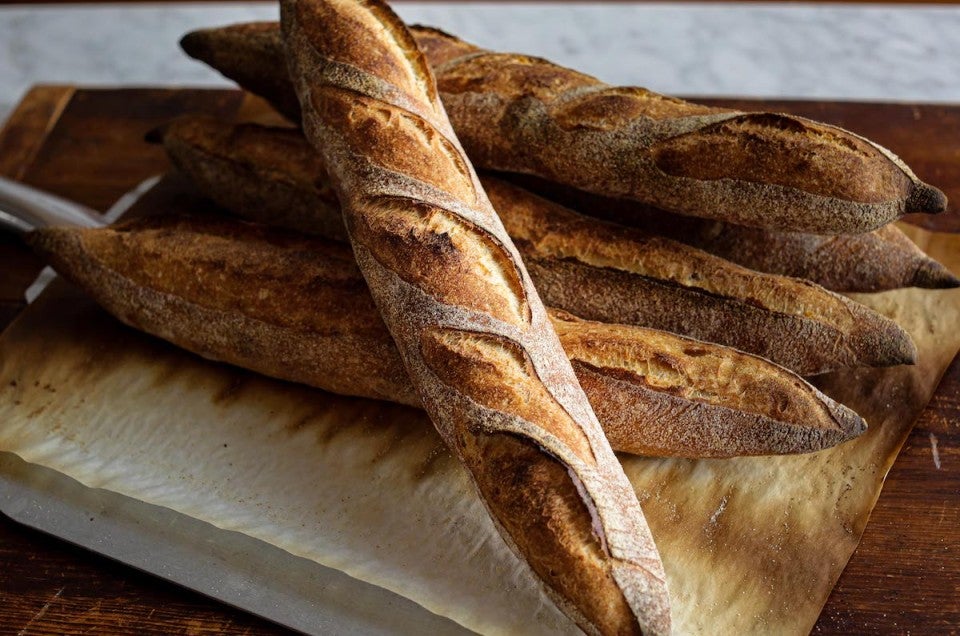This professional-looking color photograph captures five loaves of French bread, or baguettes, artfully arranged on a wooden table. The loaves, which are oblong in shape and dark brown with a burnt appearance, are sprinkled lightly with flour and bear the characteristic slits across their tops. The scene is viewed from above, with three loaves forming the base, one loaf stacked centrally on top of these, and a fifth loaf laid diagonally across the arrangement, suggesting a deliberate, rather than haphazard, placement. The loaves rest on white, slightly wrinkled parchment paper, which shows signs of being burnt around the edges. The parchment paper sits atop a rustic wooden table or cutting board, adding to the photograph’s artisanal feel. A metal pan with a silver handle is partially visible beneath, hinting at a fresh-from-the-oven setting. The lighting is such that the focus falls primarily on the diagonally placed loaf, with the top of the image appearing slightly darker to draw attention to the rich texture and details of the bread.